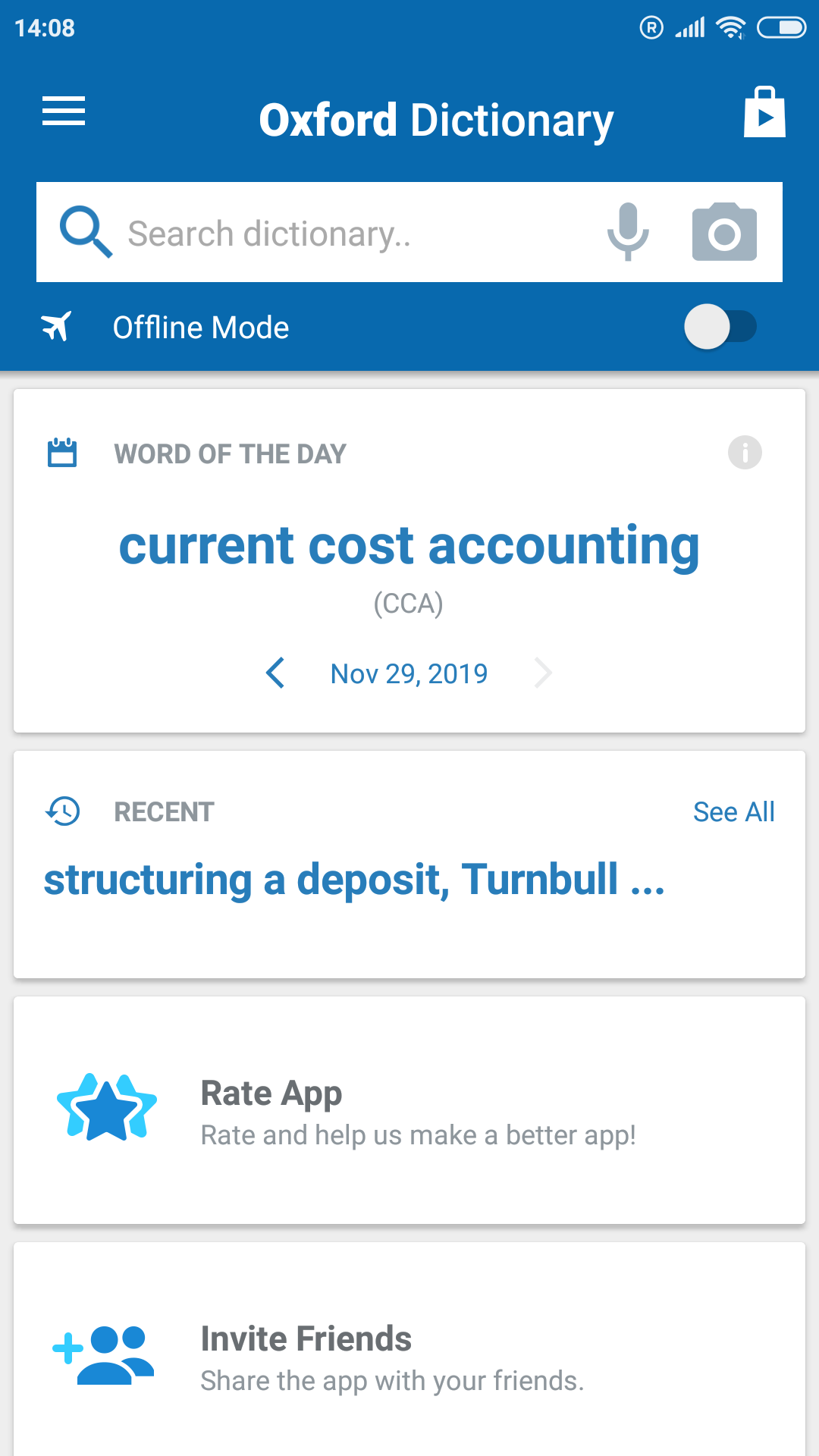### Image Description: Oxford Dictionary App Interface

The image is a vertical screenshot from a mobile device, likely an iPhone or Android, displaying the interface of an Oxford Dictionary application. The background is predominantly navy blue.

**Top Section:**
- The status bar indicates the current time as 14:08, with an "R" symbol in a white circle, three horizontal bars representing signal strength, a Wi-Fi icon, and a battery icon displaying approximately 75% charge.

**Main Interface:**
1. **App Title and Search Bar:**
   - To the right of three horizontal lines (menu icon), the words "Oxford Dictionary" are displayed in white text next to a shopping bag icon with a play button, suggesting the app could be downloaded from an app store.
   - Below this, a white search bar contains a magnifying glass icon, the placeholder text "Search dictionary" in gray, a microphone icon, and a camera icon for voice and visual searches, respectively.

2. **Offline Mode:**
   - An airplane icon and the text "Offline Mode" are positioned under the search bar, with a toggle switch beside them. The switch appears within a gray circle for activation.

3. **Word of the Day:**
   - This section includes:
     - A blue calendar icon.
     - Gray text reading "Word of the Day."
     - To the right, a lowercase "i" within a circle and "Current Cost Accounting" in blue text, abbreviated as CCA in gray beneath it.
     - Additionally, "NOV 29, 2019" with a blue left-pointing arrow indicates the date of the word.

4. **Recent Searches:**
   - A white box features a circular arrow icon resembling a refresh symbol, with "Recent" written in gray. 
   - "See all" in blue text appears to the right.
   - Below this, another search term, "Structuring a deposit, Turnbull…" is partially visible in blue text.

5. **Rating Prompt:**
   - A section with three overlapping stars—navy blue in the center, teal on the sides—entices users to rate the app. 
   - The gray text reads "Rate us," followed by smaller text urging users to "Rate and help us make a better app!"

6. **Invite Friends:**
   - At the bottom, a text box includes a teal plus sign and a navy blue icon depicting two people.
   - Gray text invites users to "Invite friends," and smaller gray text below prompts sharing the app with friends.

This interface suggests it is part of a dictionary app that allows users to search for words, view the Word of the Day, manage recent searches, rate the app, and invite friends to use it.